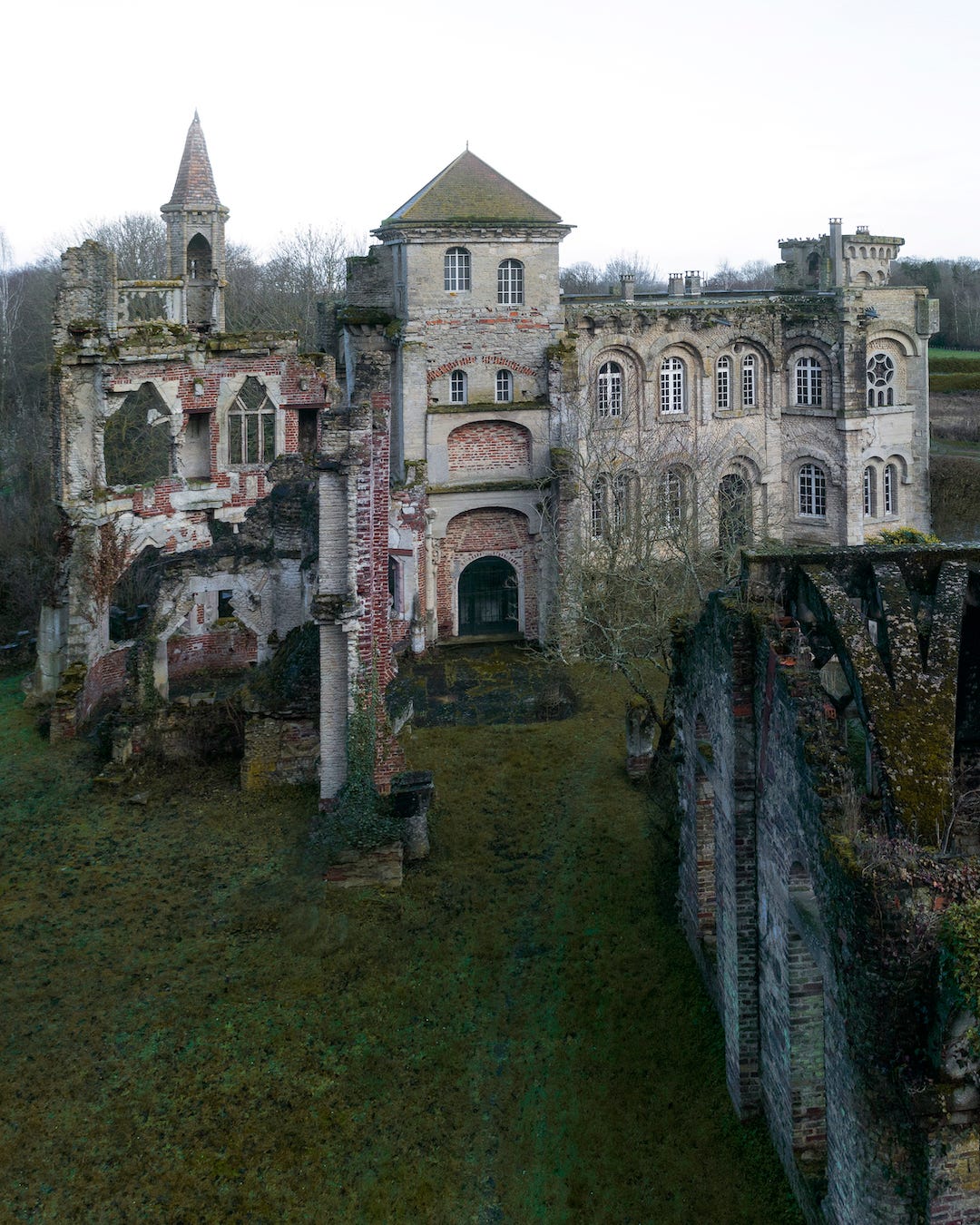This colored photograph, likely taken from a drone at a slightly overhead angle, captures the ruins of what appears to be an old, large building complex that could be a historical site, such as a former church, school, or castle-like structure. The structure is predominantly made of stone with a tannish hue, featuring a variety of heights, with sections including a medieval-style tower and a prominent archway over the entrance gate. The complex is quite run down, with visible exposed brick, and extensive moss and ivy growth covering much of the facade and rooftops. The surrounding grounds are lush but unmanicured, covered in dark green grass and dense moss. Nearby trees, both close and in the distance, add to the overgrown look of the area. In the foreground, the side of another similarly old and moss-covered building is partially visible, further emphasizing the disrepair and historical vibe of the site.